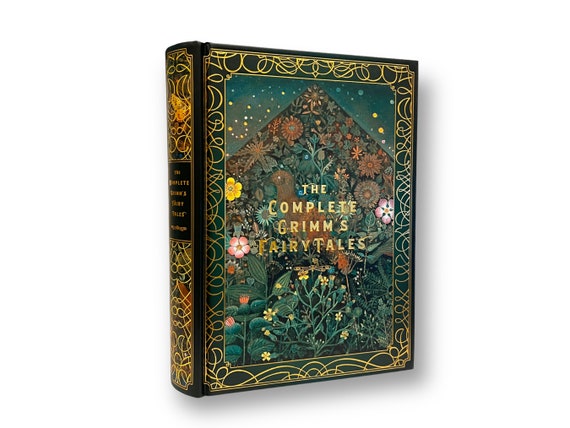This is a detailed photograph of a beautifully designed hardcover book sitting against a white background, with a slight shadow effect to its bottom and right. The book’s cover and spine prominently feature a rich, intricate filigree or Celtic-inspired gold line art along the borders. The artwork at the center of the cover boasts an abstract, medieval-inspired composition that includes a bird with a dark brown beak and light brown feathers, set amidst a vivid array of flowers and vegetation. These plants and flowers, ranging from brown and reddish to light green, pink, turquoise, and teal, are arranged in a triangular or pyramid-like form, reminiscent of natural, overgrown scenes. Surrounding this central design are small yellow, white, and light teal circles that float like stars against a blue and green-hued backdrop. The cover text, "The Complete Grimm's Fairy Tales," is prominently displayed in yellow at the center of this floral and avian vignette. Matching gold and black motifs adorn the spine, which also bears the book's title in gold lettering segmented into lines, bordered by similar golden designs. The book’s overall presentation exudes a timeless, almost magical aesthetic, fitting for the cherished tales it contains.